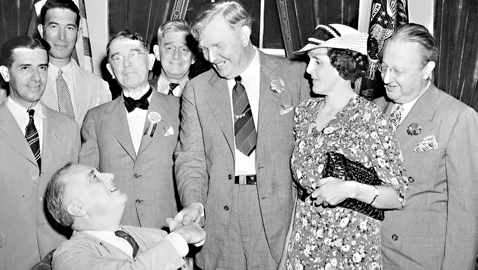The black and white photograph captures a significant moment featuring Franklin Delano Roosevelt, who is seated, likely in a wheelchair, and shaking hands with another man standing before him. Surrounding Roosevelt are six other individuals – five men and one woman – all dressed in formal attire. Most of the men are wearing suits with ties, except for one who is just in a white shirt and tie and another who sports a black bow tie. The woman stands out in a dress with a white and dark hat, accessorized by a clutch black purse tucked under her elbow. The backdrop consists of luxurious black drapes, adding to the formal and distinguished atmosphere of the gathering. The photo is clear and well-lit, offering a detailed and vivid glimpse into this historically significant encounter.